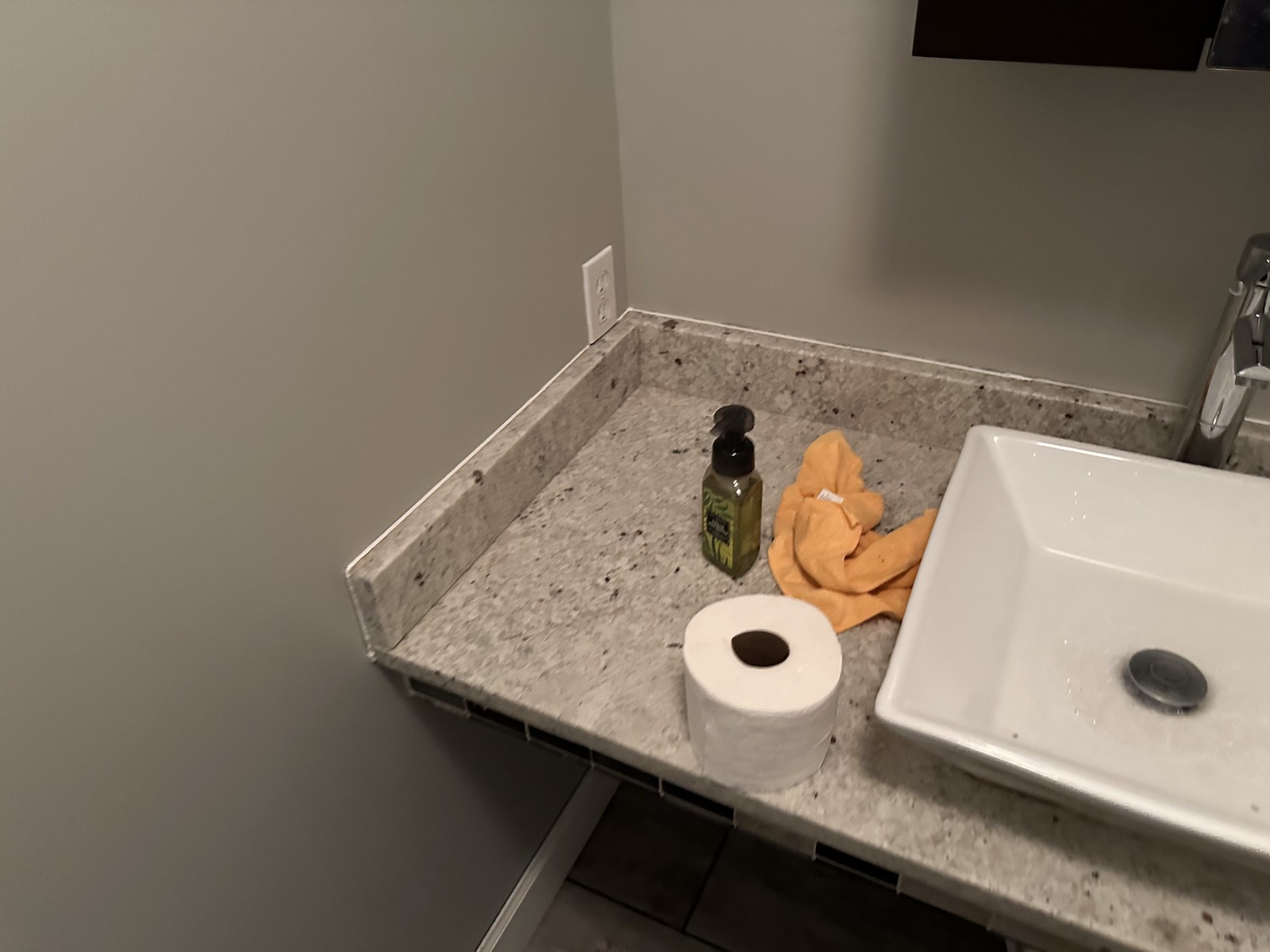The bathroom counter features a modern and sleek design. The walls are painted a grayish hue, complementing the contemporary silver, motion-activated water spigot. At the center of the tan and white Corian countertop, which is speckled with black flecks, sits a square sink with its drain positioned in the middle. A bottle of liquid soap and an orange face cloth rest on the counter, while soapy bubbles linger in the sink. A roll of white toilet paper is also placed on the countertop. Above the counter, an electrical outlet is situated just above the backsplash. Black cabinetry hangs above the spigot and sink area. The floor is tiled in a tan color, with white edging where the tiles meet the wall. It appears there is additional tiling beneath the counter, contributing to the cleanliness and cohesive look of the space.